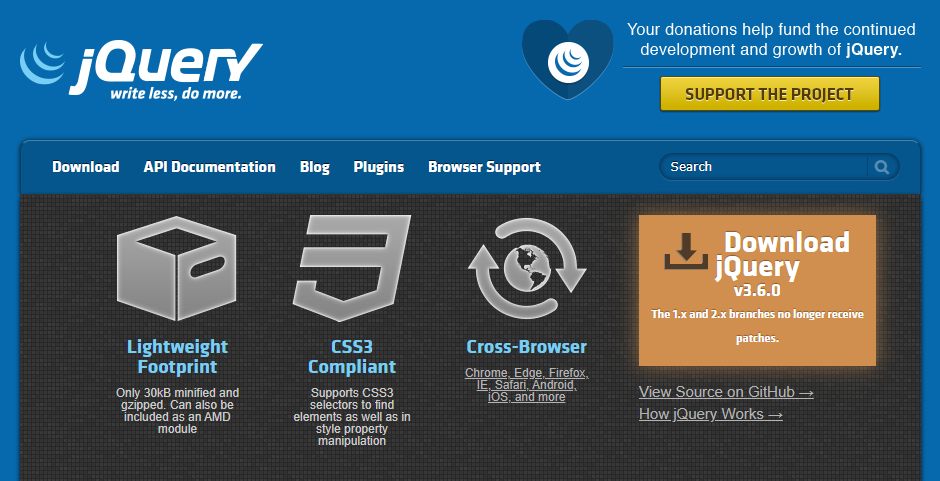This image showcases the homepage of the jQuery website. The layout features a dark blue rectangular top bar, prominently displaying three light blue, lopsided smiley faces in the top left corner. Right next to these emoticons is the stylized text "jQuery" in bold white and blue lowercase letters, with a slogan underneath in smaller writing that reads, "Write less, do more."

Further to the right on the top bar is an icon—a black or dark blue heart containing a round circle and three decreasing, half-moon shapes. Accompanying this heart icon is a white text message: "Your donations help fund the continued development and growth of jQuery." Below it, a yellow button labeled "Support the Project" with bold black letters invites users to contribute.

Continuing downward, a series of bold white menu options are listed on the left: "Download," "API Documentation," "Blog," "Plugins," and "Browser Support." Adjacent to these is a search bar.

The mid-section features a gray square icon resembling a filing box with a black interior. Below it, in light blue text, the phrase "Lightweight Footprint" appears. Another line in smaller gray text beneath elaborates: "Only 30 KB minified and gzipped. Can also be included as an AMD module." To its right, a gray symbol resembling a backward-facing 'E' with an arrow replaces the straight line. Beneath this icon, a blue text reads "CSS3 Compliant," followed by a description in gray: "Supports CSS3 selectors to find elements as well as style property manipulation."

Further right, a gray icon depicts two arrows forming a circle with a globe inside. Below it, light blue text reads "Cross-Browser," and beneath, smaller text lists compatible browsers and platforms: "Chrome, Edge, Firefox, IE, Safari, Android, iOS, and more."

Finally, the bottom right section features a large brown button with bold white text that states, "Download jQuery v3.6.0." An additional note specifies, "The 1.x and 2.x branches no longer receive patches."